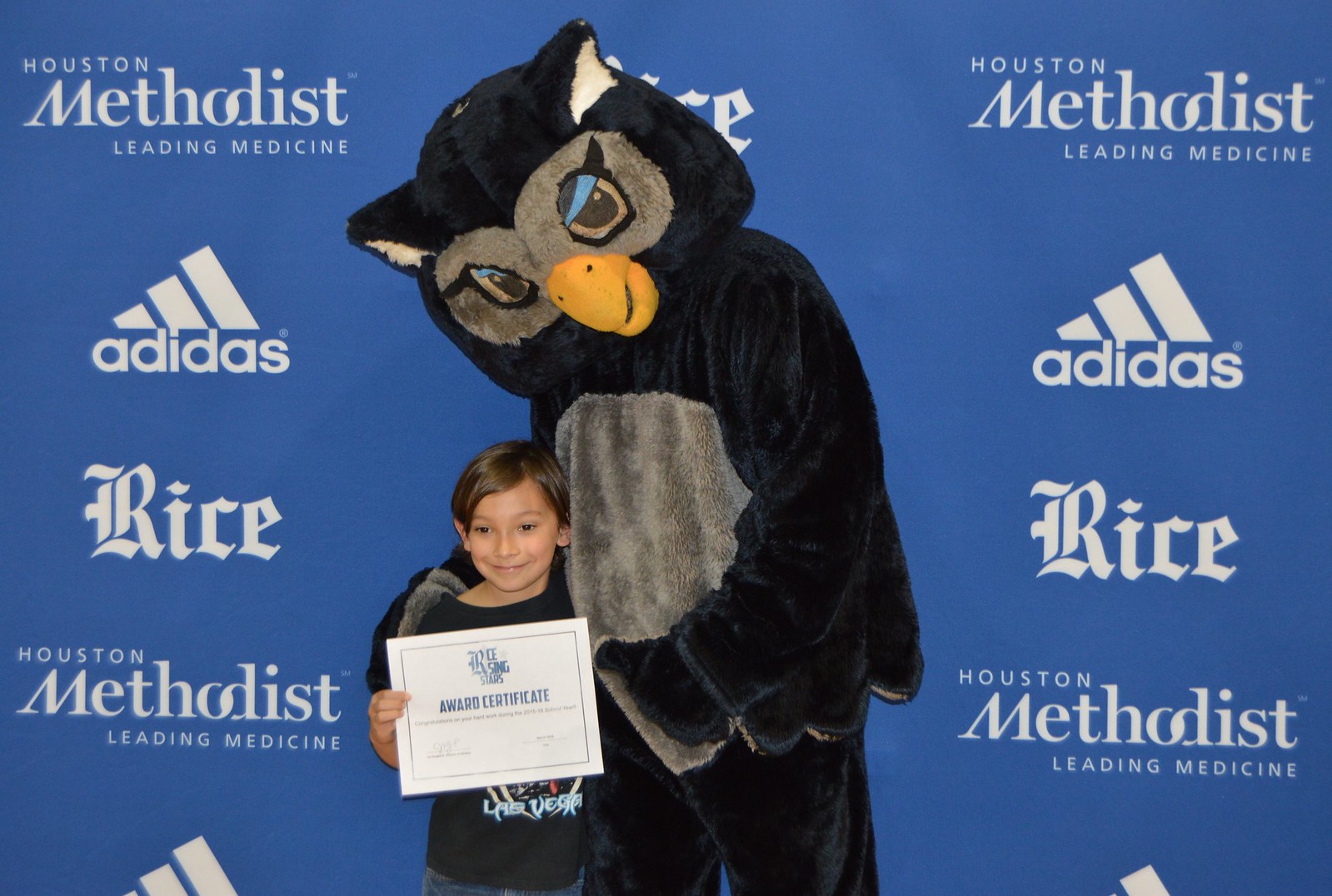In this photo, a young boy is smiling and holding an award certificate in his right hand. He is wearing a black t-shirt and standing in front of a blue backdrop adorned with white logos, including those of Houston Methodist Leading Medicine, Adidas, and Rice University. Next to him stands a person dressed as Sammy the Owl, the mascot of Rice University. The person in the owl costume has their right arm around the boy's shoulder, embracing him in a supportive and celebratory manner. Behind them, the blue backdrop serves as a wall adorned with text representing various companies and sponsors of the event. The boy, appearing happy, poses proudly with his award certificate while the owl-costumed figure supports him warmly.